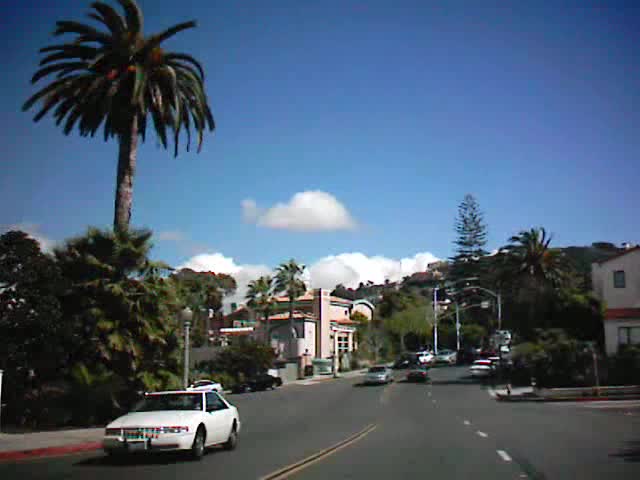In this street-level photograph, likely taken from within a car, we find ourselves on a busy four-lane road, comprising two lanes in each direction. The center of the road is marked by a clear double yellow line, while a broken white line delineates the lanes. Dominating the bottom left-hand corner is a white car, set against the backdrop of lush palm trees and a sidewalk featuring a red curb. Further in the distance, various elements come into view: an architectural building adorned with multiple windows, additional palm trees, and five more vehicles under the subtle watch of tall light poles. To the far end of the scene, a mountain or hill provides a scenic background. Shifting attention to the right, a beige two-story home with contrasting red trim stands prominently. The house showcases two visible windows and is also bordered by a sidewalk, accompanied by an illegible road sign.